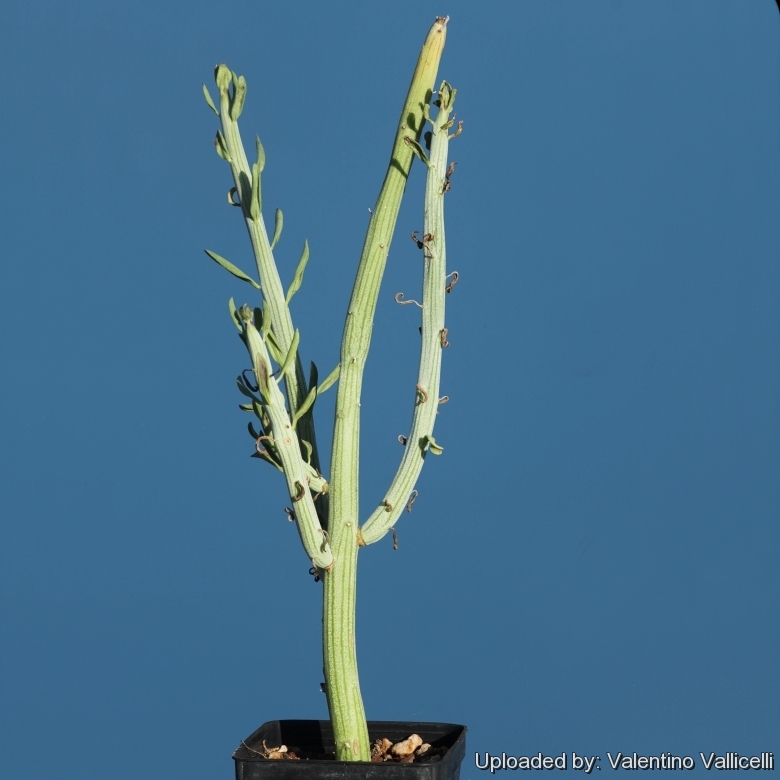This is a highly detailed photograph of a cactus-like green plant set against a dark blue background, with white text at the bottom right reading "Uploaded by Valentino Vallicelli." The plant is housed in a small black plastic pot filled with rocks. It features one main thick, light-green stalk adorned with striations that give it a celery-like appearance. Extending from this main stalk are three distinctive sprouts of varying sizes: the longest on the right, a very short one on the lower left, and another longer one positioned slightly higher up. Each sprout displays emerging leaves—some newly unfurled and others still developing. Additionally, there are small, round, spiky leaves sprouting from the main stalk, with some showing signs of decay. The overall composition highlights the rich textures and vibrant hues of the plant within its minimalistic yet striking setting.